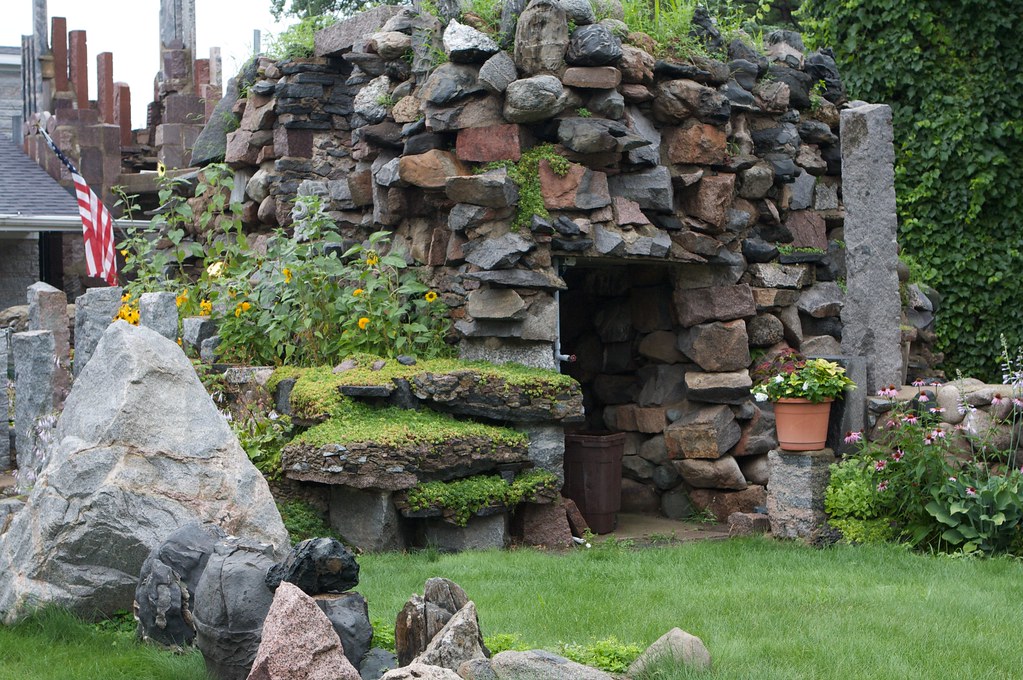This color photograph showcases a large stone structure, reminiscent of a tomb or cave, built from variously shaped dark gray, brown, and reddish stone blocks stacked together. The central feature is a square opening that serves as an entrance, contributing to its tomb-like appearance. To the right of this entrance, a ceramic planter filled with yellow flowers and green leaves adds a splash of color. Ivy covers a wall adjacent to the structure, with moss-covered boulders and other stone elements like pillars seen in the background. The area in front of the structure is covered with short green grass, and additional rocks and boulders, some moss-covered, can be found to the left. In the top corners of the image, you can see dark green ivy and gray-brown skyscrapers in the distance, and an American flag is visible behind the structure.